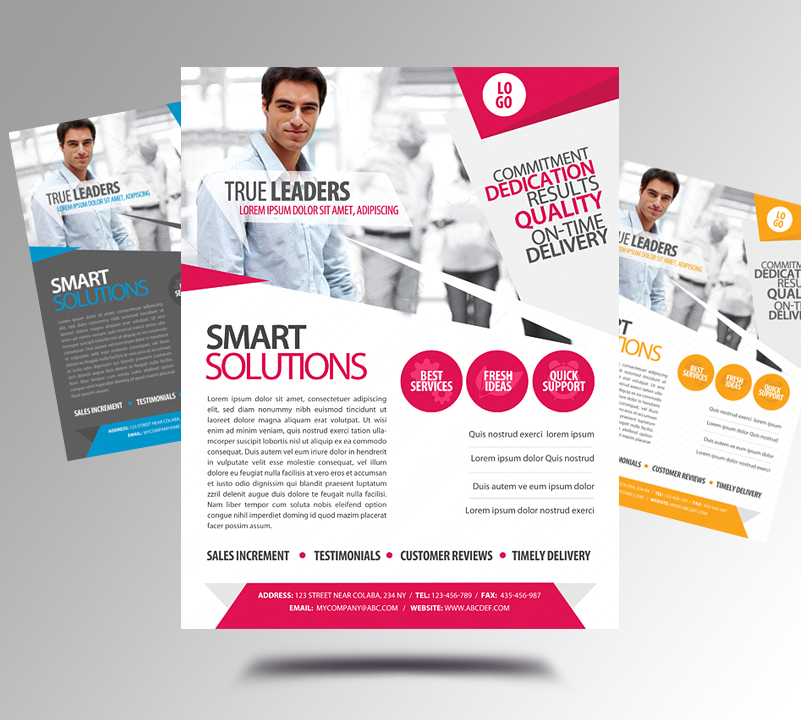The image displays a set of three mock-up flyers, each featuring a man with dark hair in a light blue button-down shirt, smiling at the camera. The central flyer is predominantly white with pink accents, while the ones on the left and right are variations in blue and darker gray, and yellow and gray, respectively. The headline on each flyer reads "True Leaders," followed by placeholder text "Lorem Ipsum" in pink.

The flyers have a consistent layout: 

- The man's image appears in the upper left corner, with his body slightly turned to the right.
- Beside the image, a pink (or red in some descriptions) banner with "LOGO" in a white circle is placed.
- Below the banner, a series of words in black or pink text reads: "Commitment, Dedication, Results, Quality, On-Time Delivery."

In the bottom half:
- The phrase "Smart Solutions" is split into black (Smart) and pink (Solutions) text.
- Beside this, there are three pink circles labeled "Best Services," "Fresh Ideas," and "Quick Support."
- Below the circles, lines of small placeholder text (Lorem Ipsum) are separated by horizontal lines.
- The bottom of each flyer features the phrases "Sales Increments," "Testimonials," "Customer Reviews," and "Timely Delivery," separated by pink bullet points.
- At the very bottom, a pink color block contains placeholder address information in white font.

Overall, the flyers are visually unified in layout and structure, differing mainly in their color schemes.